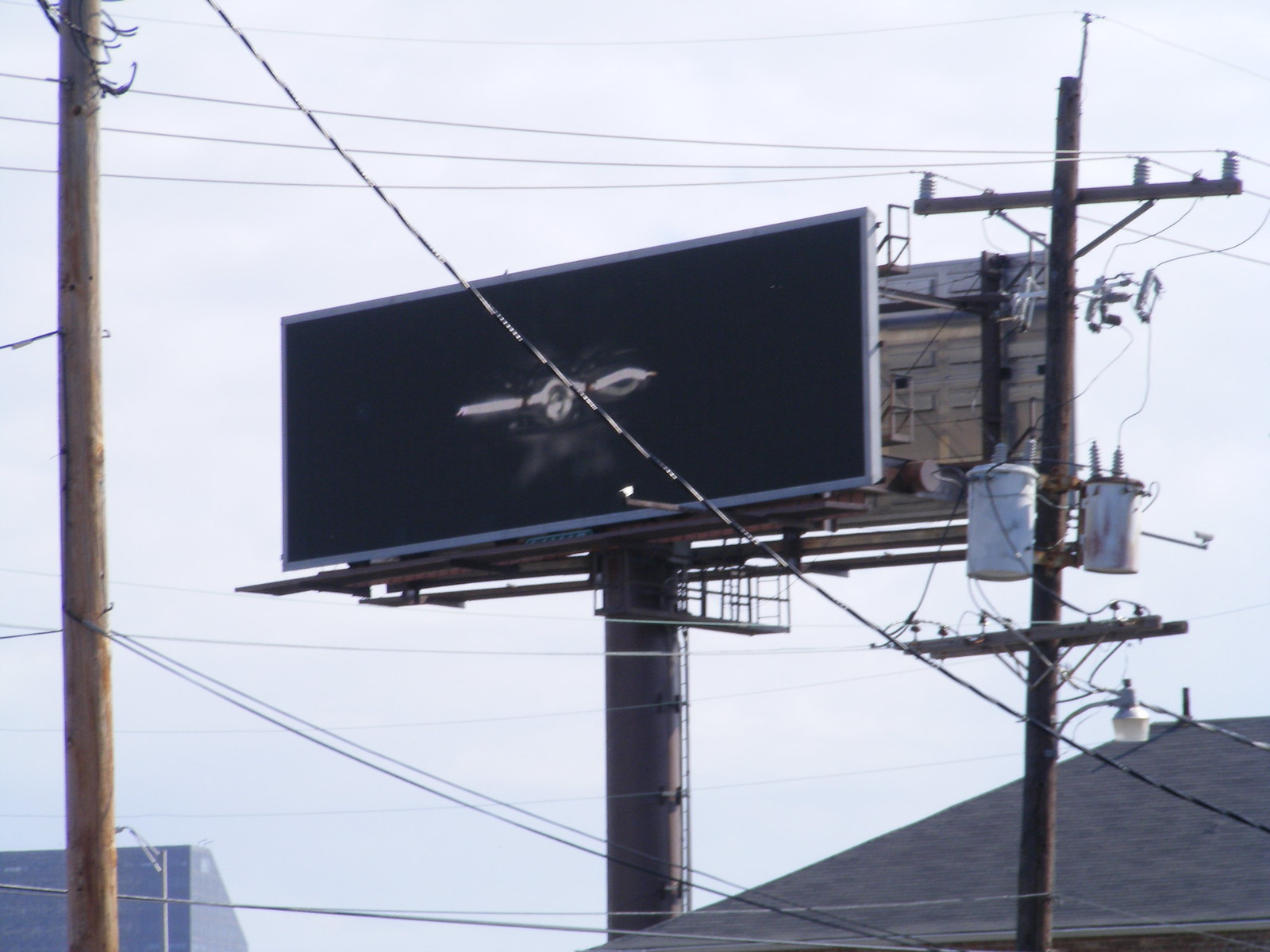The image showcases a dual-billboard setup mounted on a single, large, dark-colored post under an overcast gray sky. The primary billboard features a black background emblazoned with an enigmatic gray object in the center. This object appears as a sequence of shapes: a gray line, followed by a roundish gray form, and ending with an outline resembling an arrowhead. The true nature or purpose of this object remains unclear. Behind and partially obscured by the primary billboard, a second billboard is visible from the rear, lacking any visible content from this angle. Below the billboards, a gated platform is present, likely designed for maintenance personnel to stand between the billboard bases. The image is crisscrossed with utility lines running diagonally and horizontally, anchored by at least two utility poles in the foreground. Additionally, the scene includes varied architectural elements with a blue-roofed structure and another building topped with a dark-colored roof, all under a blanketing layer of gray clouds.